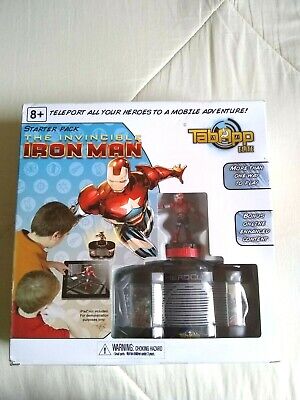This color photo captures a boxed Iron Man game set on a white quilted comforter, resembling a mattress. The game box, prominently labeled "Starter Pack: The Invincible Iron Man," features Iron Man in a dynamic flying pose, adorned in his iconic red and gold suit. The box also highlights the text "8 Plus, Teleport all your heroes to a mobile adventure," and includes branding in the top right corner that reads "TabApp" in yellow. Additionally, there is a cautionary note about a choking hazard at the bottom. The packaging shows an exposed clamshell area revealing a miniature Iron Man figure inside. To the left, an image depicts a father and son engaging with the game on an iPad, emphasizing the interactive mobile adventure aspect.